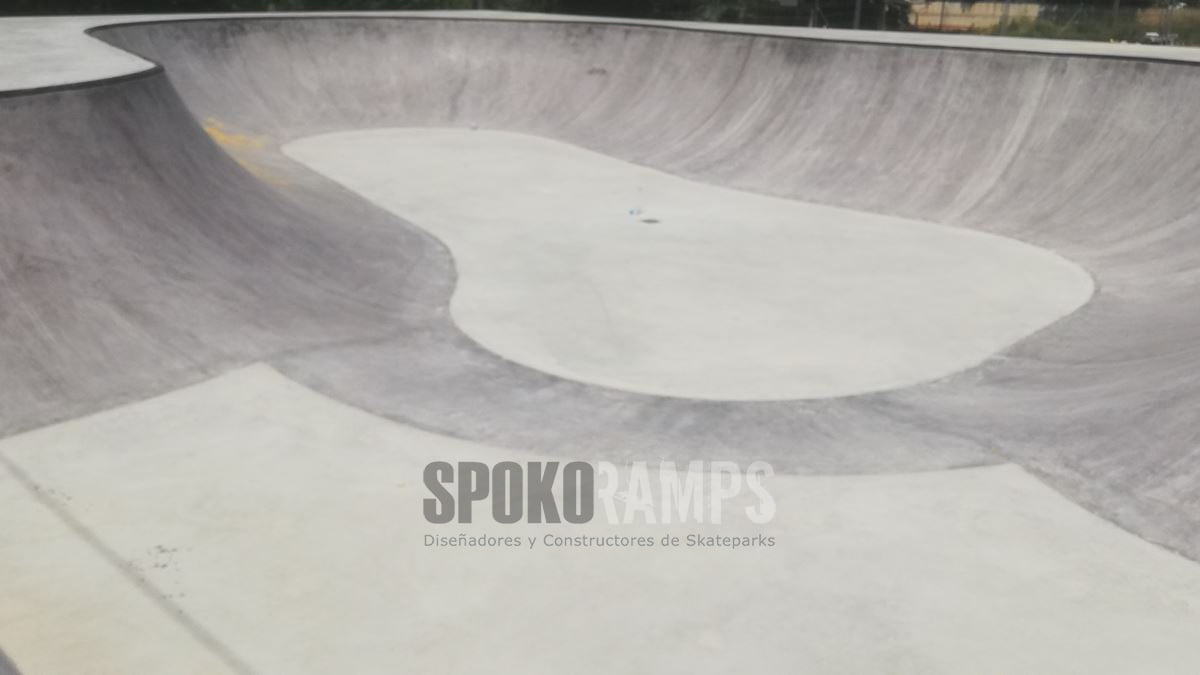The image depicts an outdoor skate park photographed during the daytime, likely an older, slightly faded rectangular photograph approximately six inches wide and four inches tall. The skate park, which features curved and rounded concrete areas, is currently empty. The structure is constructed primarily of light gray and dark gray concrete, with the darker gray highlighting the curved and inclined sections, while the flat surfaces are in a lighter shade of gray. 

In the bottom center of the photograph, in bold gray text, appears the name "Spoko" followed by the word "Ramps" in opaque white print. Below this, in smaller light gray text, the phrase "Descendores y Constructores de Skate Parks" is visible. This area of the image also includes minimal background details, with some indistinct elements visible in the top right corner. The composition emphasizes the emptiness and the unique architecture of the skate park, revealing the smooth, rounded bowl area where skateboarders would typically perform their tricks.